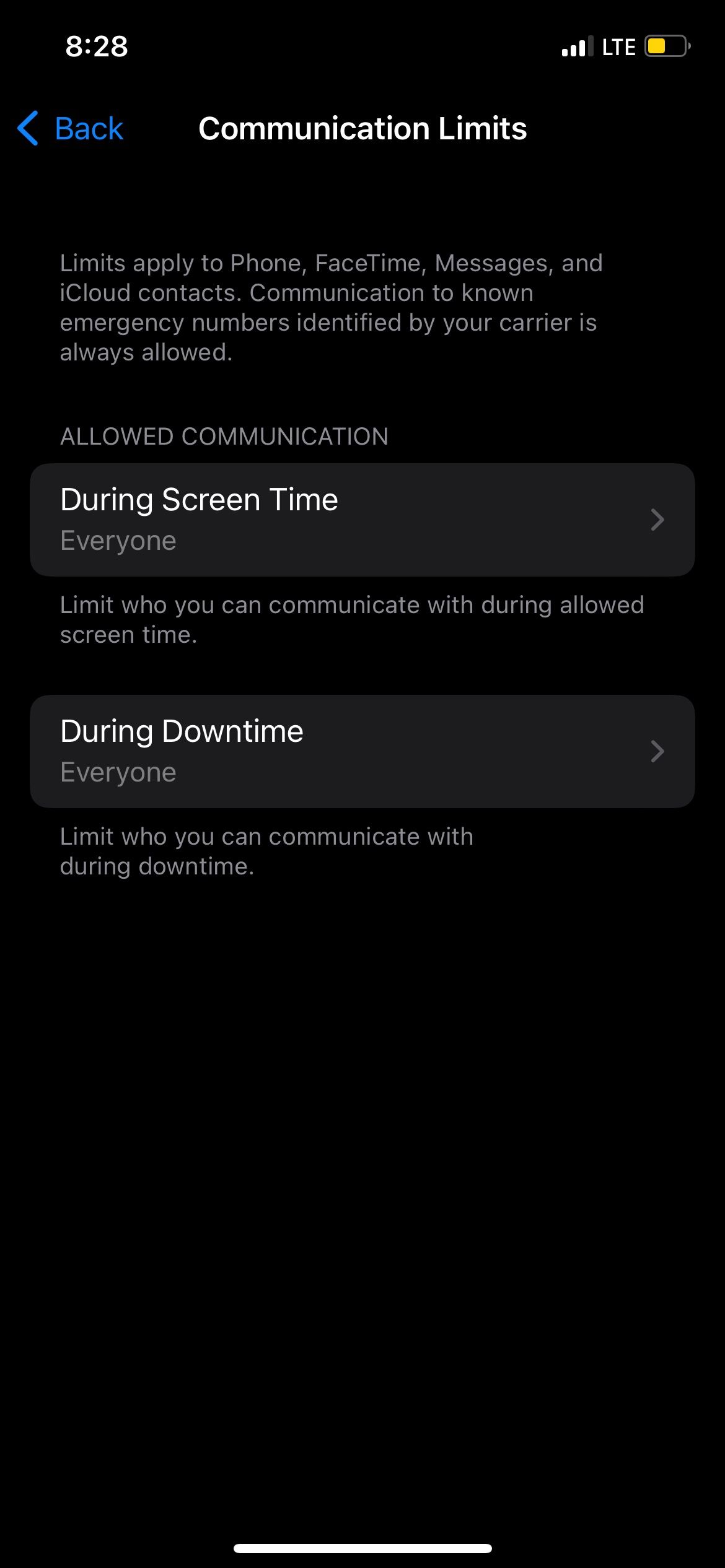This image is a screenshot displayed in portrait mode with a black background. In the upper left-hand corner, the time is shown as "8:28", while the upper right-hand corner displays a half-charged battery icon in yellow. 

Below this, the left side features a blue "Back" button, and centrally, in bold white text, the heading reads "Communication Limits". A gray subtitle explains, "Limits apply to phone, FaceTime, Messages, and iCloud contacts. Communication to known emergency numbers identified by your carrier is always allowed."

The next section is titled "Allowed Communication." There are two main options displayed as gray buttons with bold white text. The first button reads "During Screen Time" with a gray subtitle underneath that says "Everyone." This option allows you to limit who can communicate with you during allowed screen time. 

The second button reads "During Downtime" with a gray subtitle underneath that says "Everyone." This option allows you to limit who can communicate with you during downtime. Both options end with right arrow menus indicating further expandable settings for additional details.

This screenshot pertains to setting communication limits on a device, specifying who is allowed to contact you during screen time and downtime.